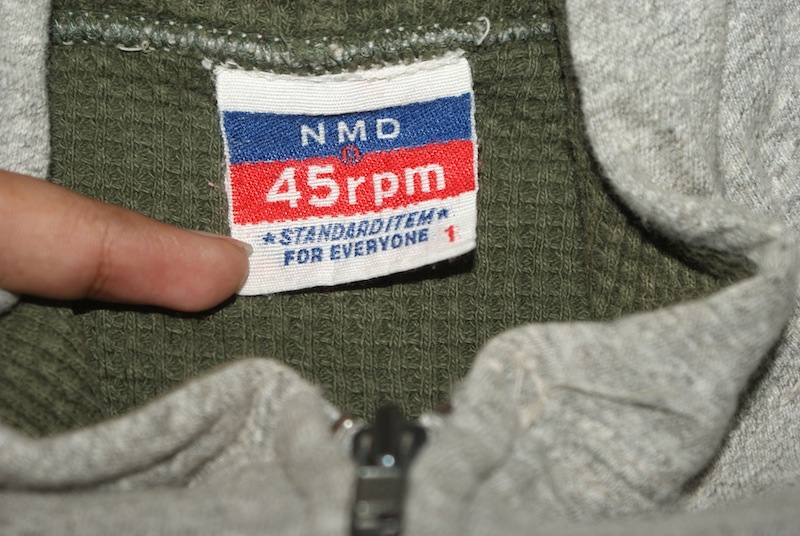This photograph captures the detailed view of the collar of a thick-lined winter jacket, predominantly gray in color with a wool-like texture. The interior of the jacket features a unique square-sewn texture, enhancing its warmth and style. A black zipper runs down the front of the jacket. From the left side of the image, a finger points towards a tag attached to the collar. The white tag, bordered in blue and red, reads "NMD" and "45 RPM" respectively. Below, in blue print, it states "standard item for everyone" followed by the number "1".